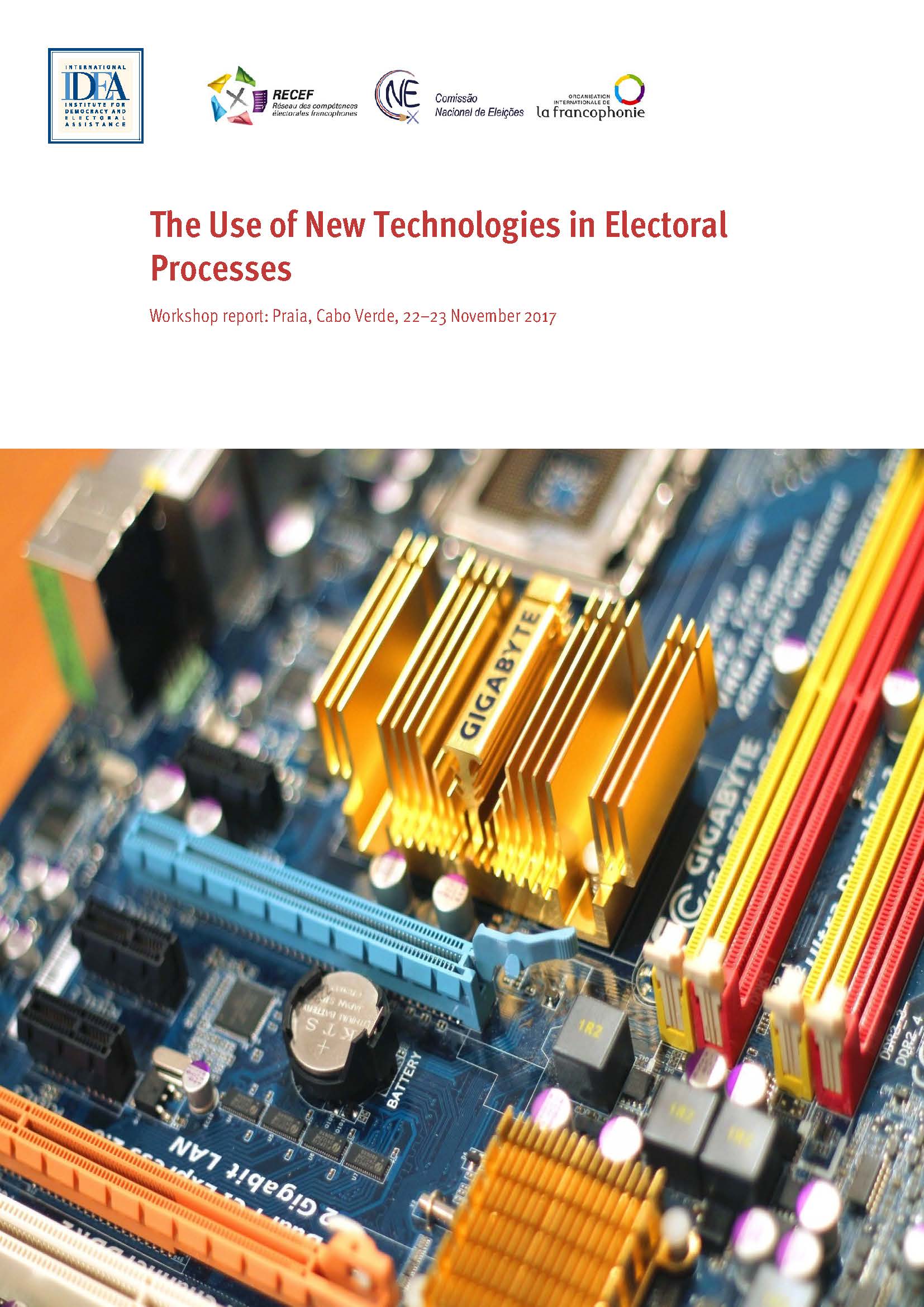This detailed square color photograph, taken from above on a white background, showcases a blue circuit board adorned with various electronic components. Prominently placed in the center is a gold heatsink labeled "Gigabyte" in black print. The board features an array of square and rectangular chips, many of which are aligned vertically within the frame. Notably, there's a rectangular pattern of over a dozen square golden plates arranged in a row, while the right edge of the board is populated by eight elongated rectangular chips, and rows of red and yellow components. The top of the image features logos, including one identifiable as "IDFA", followed by three others. Below the logos, bold red text reads "The Use of New Technologies in Electoral Processes Workshop Report, Pralokkava Verde, 22-23 November 2017." The circuit board has intricate black runs interspersed with white print, with visible labels such as “Gigabyte L-A-N.” The vivid hues of gold, blue, yellow, and red further enhance the intricacy and complexity of the motherboard.